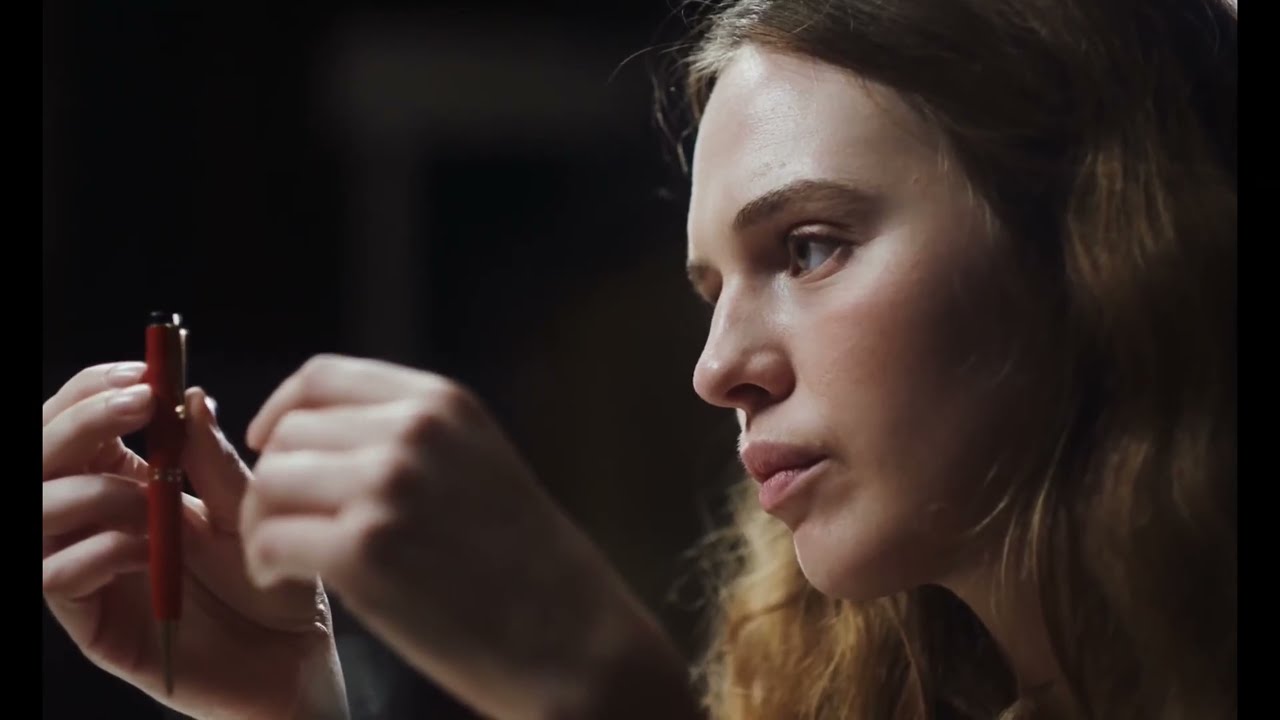The photograph features a light-skinned woman with wavy, light golden-brown hair and brown eyes, staring intently to the left. She is holding a red pen with a black top in her right hand, with her short, unpainted nails visible. Her face is prominently shown on the right side of the image, capturing a focused expression as she examines the pen. The dark, black background hints at being indoors, with strips of black running down both sides and a blurry white pole in the distance. The lighting source from the left illuminates her forehead and nose, highlighting her features. The overall color palette and the composition suggest the woman is of Caucasian descent, likely of European origin, and the setting is a close-up, detailed study of her contemplative moment with the pen.